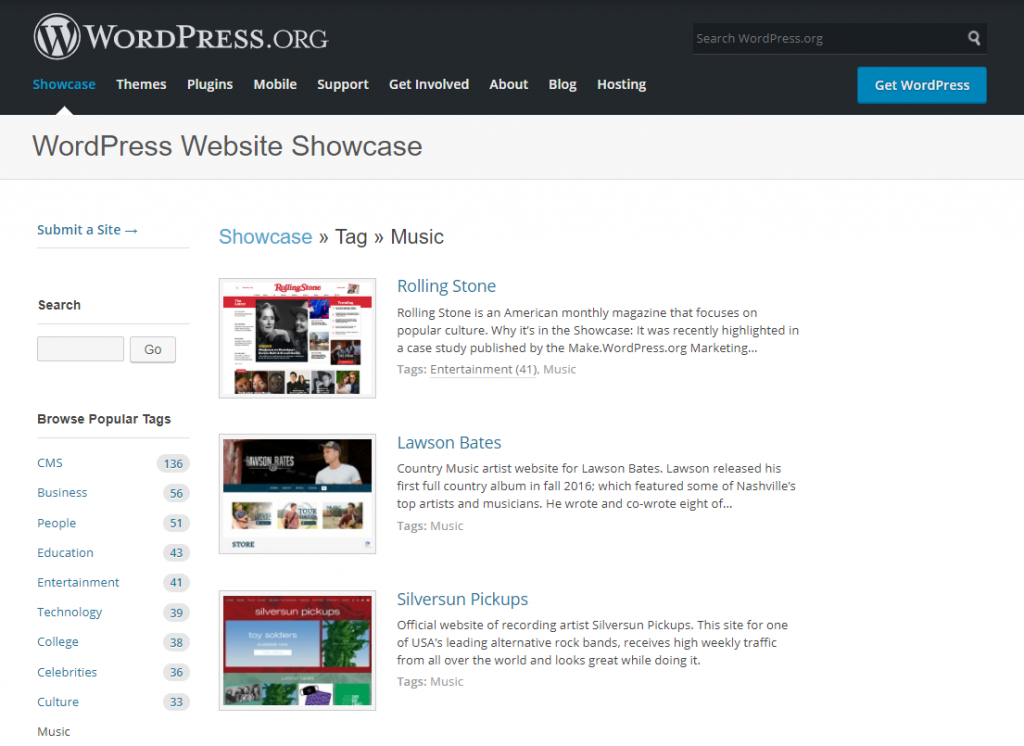This is a detailed description of the image in question, carefully formulated into a comprehensive caption:

---

The top of the webpage features the WordPress.org header, including a search bar with options for "Showcase," "Themes," "Plugins," "Mobile," and "Support." Below this, there is a blue rectangle button prompting users to "Get WordPress." The text "WordPress Website Showcase" indicates the section, encouraging users to submit their own sites. A right arrow leads to further showcase tags and categories.

The next section highlights the "Rolling Stone" magazine, identifying it as an American monthly publication focused on pop culture. The magazine's showcase was recently featured in a case study published by The Make.

Featured artist Austin Bates is spotlighted with his country music website, noting his first full album released in 2016 and his introduction to Nashville's top five list.

Additionally, the official website for Silver Sun Pickups, a leading alternative rock band in the USA, is highlighted. It is recognized for its high weekly traffic from global visitors and its attractive design.

The footer includes tags such as "Music," "CMS," "Business," "Entertainment," "People," "Education," "Technology," "College," "Celebrities," "Culture," and "Music Background."

---

This expanded and cleaned-up version describes all elements accurately, providing a well-rounded view of the image.